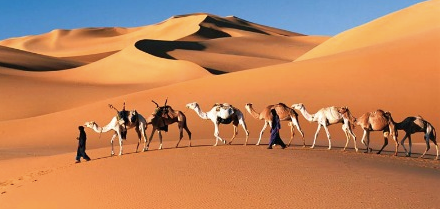The image captures an expansive desert landscape dominated by towering sand dunes stretching into the horizon. In the midst of this arid expanse, two men clad in traditional dark Bedouin attire are seen as mere silhouettes, guiding a caravan of seven camels. The camels, uniformly white and tan, walk in a single file, each carrying supplies. The front two camels appear to be fitted with saddles, though the men lead the caravan on foot. Trailing behind them in the soft, brownish-tan sand are distinct footprints and hoof prints, lending a sense of movement and journey. Above, a vibrant, cloudless blue sky forms a striking contrast with the golden dunes. Shadows cast on the rippling ridge lines of the dunes emphasize their imposing height and texture. The scene is imbued with a serene yet awe-inspiring beauty, with no indication of other life for miles, evoking the timeless solitude of the Sahara Desert.